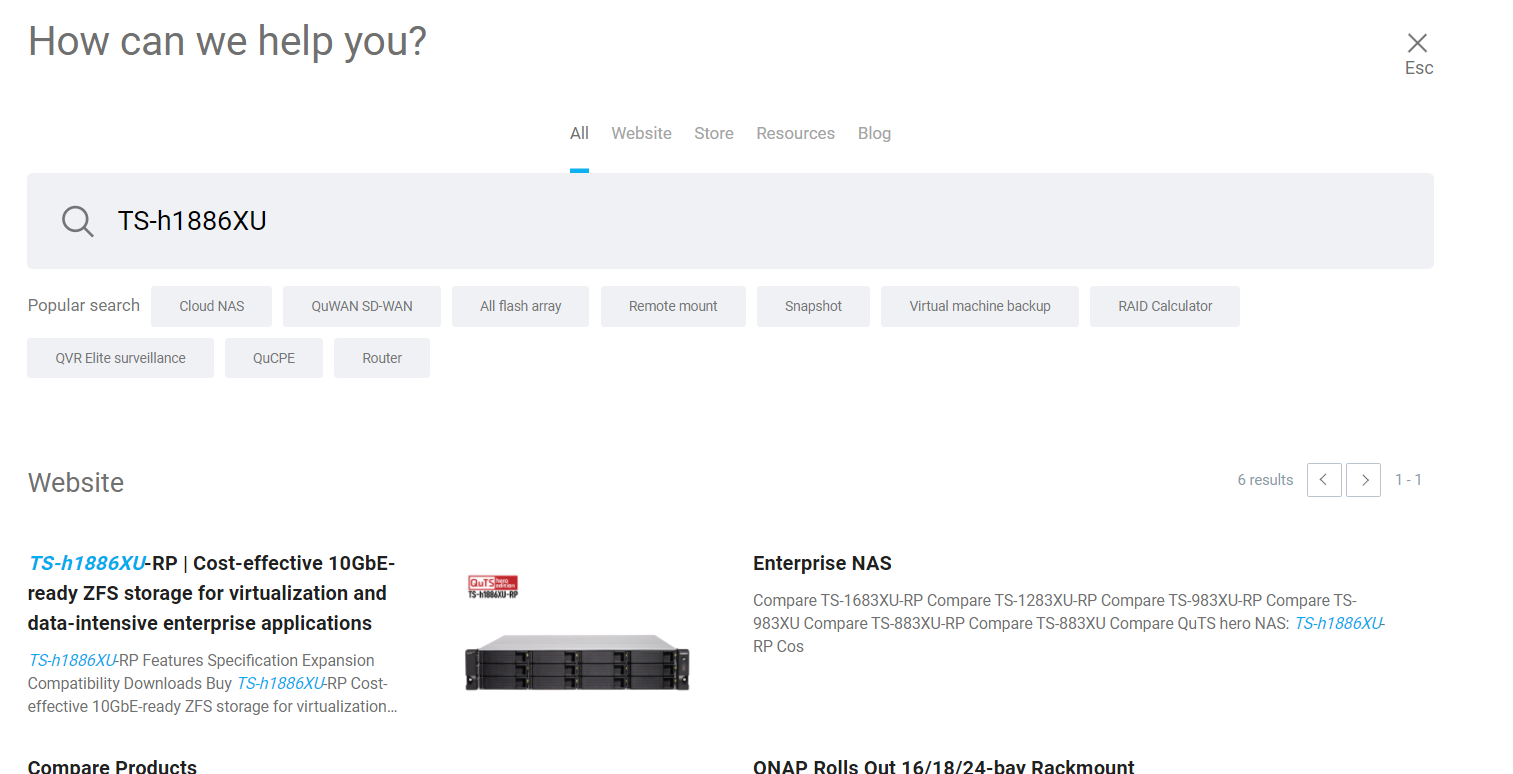The image features a detailed webpage with the top background split into white and black sections. On the white section, the text "How can we help you?" is displayed in black. The black section contains a small "X" icon. Below this, there is a capital letter "E" followed by "SC," and an underlined word "ALL" in blue, all in black font except for the blue underline.

Further down, the webpage has navigation links reading "Website," "Store," "Resources," and "Blog" in black font, with "ALL" in bold compared to the others. Underneath, there is a gray text box with a black magnifying glass icon next to it, inside which someone has typed "TS-H1886XU" in all capital letters. A "Publisher Search" button is adjacent to this text box.

Below the search bar, there are a series of small gray boxes with dark gray text that lists terms such as "Cloud," "NAS," "Q Quan," "SD Wand," "FlashArray," "Remote Mount," "Snapshot," "Virtual Machine," "Backup," "RAID Calculator," "QVR," "At Least," "Surveillance," "QPC QCP," and "Router."

In black text, it reads "Website," followed by a blue text "TS-H1886XU." Then, it switches back to black text, with "—RP" and continues in the same font, "Cost-effective 10 GbE ready ZFS storage for virtualization and data-intensive enterprise applications."

Additional sections labeled "Features," "Specification," "Expansion," "Compatibility," and "Buy It" follow. The phrase "Cost-effective 10 GbE ready ZFS storage for virtualization..." trails off with an ellipsis. There's also a prompt to "Compare Products." Towards the bottom, a black box states "QNAP rolls out 16/18/24 bay rack mount," signaling new product offerings.